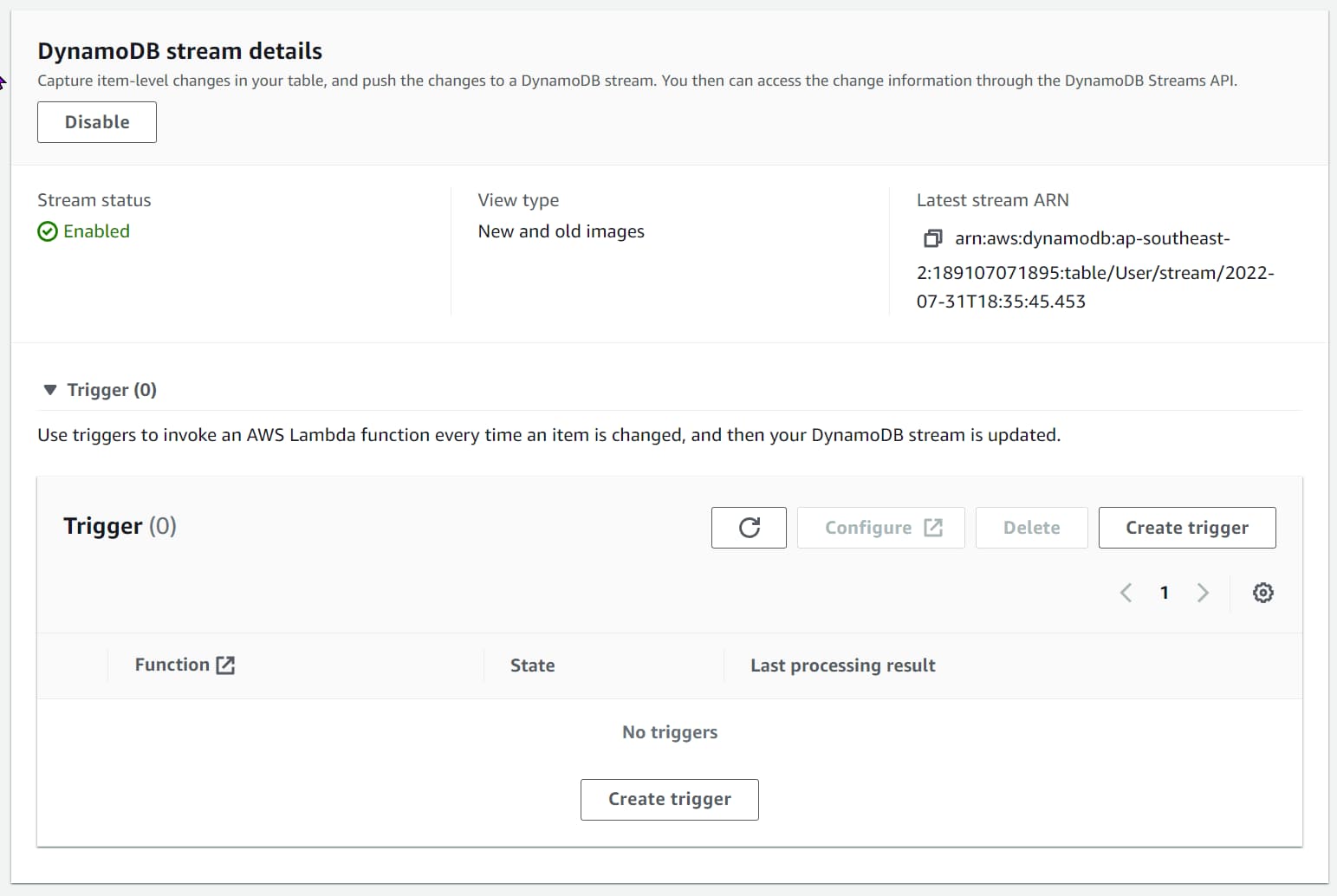**DynamoDB Stream Details Interface**

The image is a screenshot of a webpage or program interface displaying detailed information about DynamoDB Stream Details. 

**Header:**
- At the very top, centered within a light gray strip that spans horizontally, is the title "DynamoDB Stream Details" rendered in bold black text.
- The background of the page is predominantly white.

**Top Section:**
- Directly beneath the title, in tiny letters, the interface explains: "Capture item level changes in your table and push the changes to a DynamoDB Stream. You then can access the change information through the DynamoDB Stream API."
- Below this description, a button labeled "Disable" is present, giving the option to disable the DynamoDB Stream.

**Middle Section:**
- This part of the page has a continuation of the white background.
- It provides several key pieces of information in a list format:
  - **Stream Status:** Displayed as "Enabled," highlighted in green with an accompanying green checkmark and a circle symbol.
  - **View Type:** Stated as "New and Old Images."
  - **Latest Stream ARN:** Followed by a detailed ARN string that starts with "arn:aws:" and includes a long sequence of additional characters and numbers.
  
**Bottom Section:**
- A section for "Triggers" is defined, though it currently indicates zero triggers with a parenthetical (0) and a downward-pointing arrow. 
- This is explained further: "Use triggers to invoke an AWS Lambda function every time an item is changed and then your DynamoDB Stream is updated."
- As there are no triggers set up, a line states "No triggers" and below it, a button offers the option to "Create a Trigger."

**Footer:**
- The bottom-most part of the page displays a light gray bar, similar to the one at the top but with no additional content.

Overall, the interface provides comprehensive information on the current status and configuration of the DynamoDB Stream, allowing users to manage and monitor their stream and trigger settings efficiently.